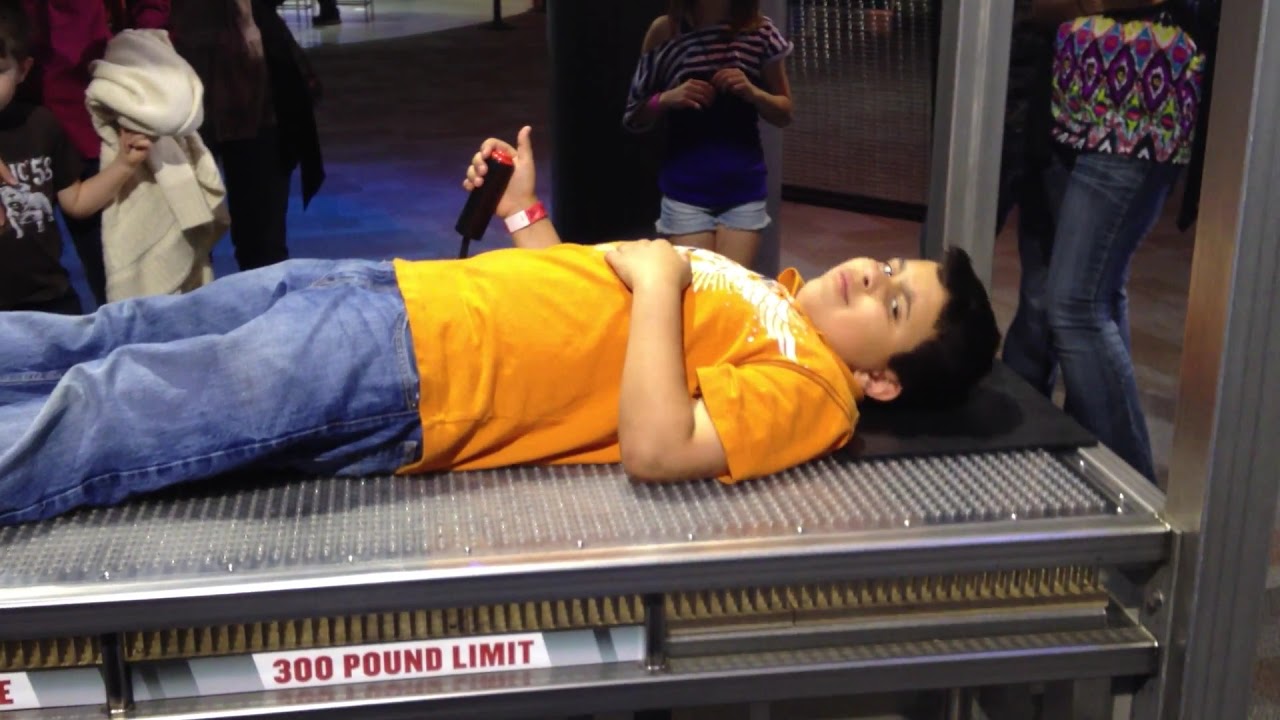A young boy, roughly 12 to 13 years old, is lying on his back on a peculiar contraption that resembles a bed of nails or a large metal scale, indicated by a noticeable red rectangular label stating "300 pound limit" on its side. He is wearing a mustard-colored, short-sleeved collared shirt with a white wing-like design on the front and blue denim pants. In his right hand, he holds a black controller with a red button, his thumb poised as if about to press it, projecting a sense of anticipation. His left hand rests over his chest, and he looks directly at the camera with a slightly mischievous expression. Surrounding him is a small group of onlookers: one person's lower half is visible, clad in jeans and a multicolored shirt with the word "Diamonds" and various shapes on it. Another figure in the group is wearing denim shorts and a blue shirt, while a third person holds a white sweatshirt. Additionally, there is a small boy dressed in black and another individual in a brown outfit present in the background, all seemingly fixated on the boy on the metal setup.